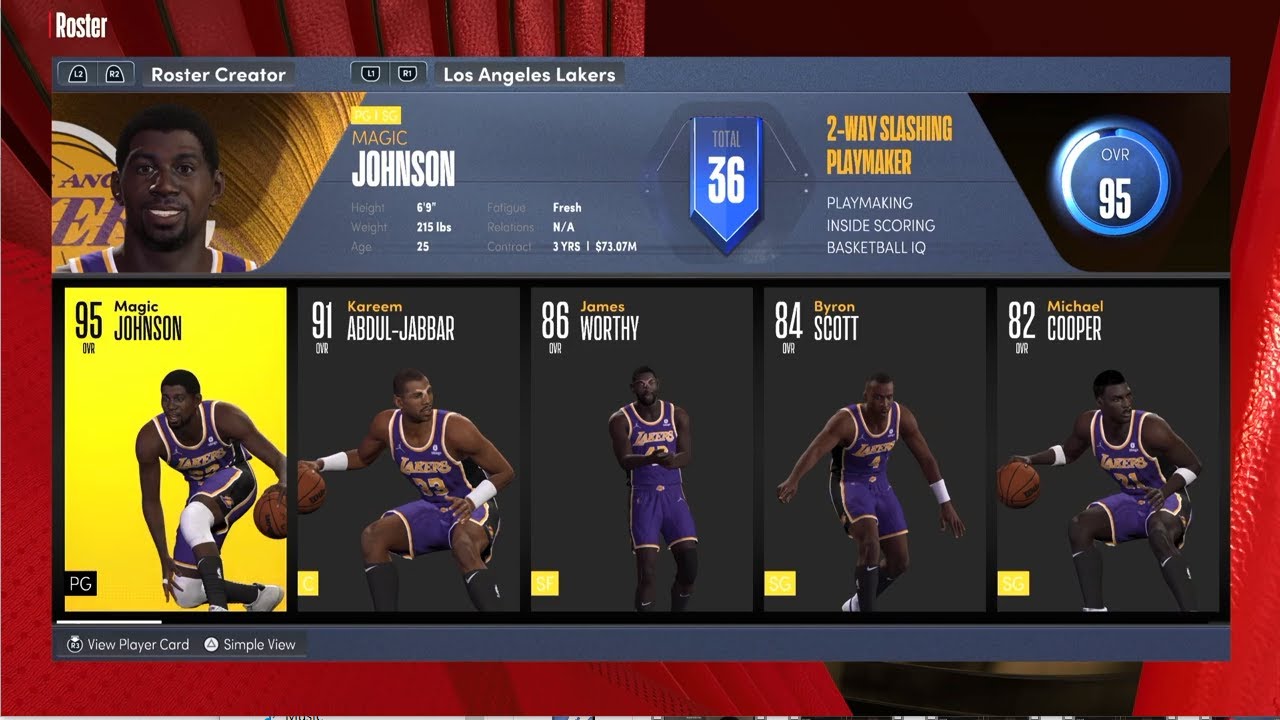This screen capture from an NBA video game showcases the roster management interface. In the upper left corner, the word "Roster" is prominently displayed in white font against a red, leathery textured background. Centered on the screen is a large blue box detailing the current roster for the "Los Angeles Lakers."

At the top of the blue box, the team name "Los Angeles Lakers" is clearly indicated. Below, detailed information about Magic Johnson is provided: he stands 6'9" tall, weighs 215 pounds, is 25 years old, is currently "Fresh" in terms of fatigue, and has a contract lasting 3 years worth $73.07 million. A banner labeled "Total 36" appears, followed by his player archetype and skills, which include "Two Way Slashing Playmaker," "Playmaking," "Inside Scoring," and "Basketball IQ." On the right-hand side, a blue circle denotes his overall rating of 95.

To the left of the blue box, a digital rendering of Magic Johnson is shown. Below this image, the starting lineup for the Lakers is listed, featuring:
- Magic Johnson: Overall 95
- Kareem Abdul-Jabbar: Overall 91
- James Worthy: Overall 86
- Byron Scott: Overall 84
- Michael Cooper: Overall 82

Each player's name and overall rating are accompanied by their respective video game avatars, completing the detailed representation of the Los Angeles Lakers roster.